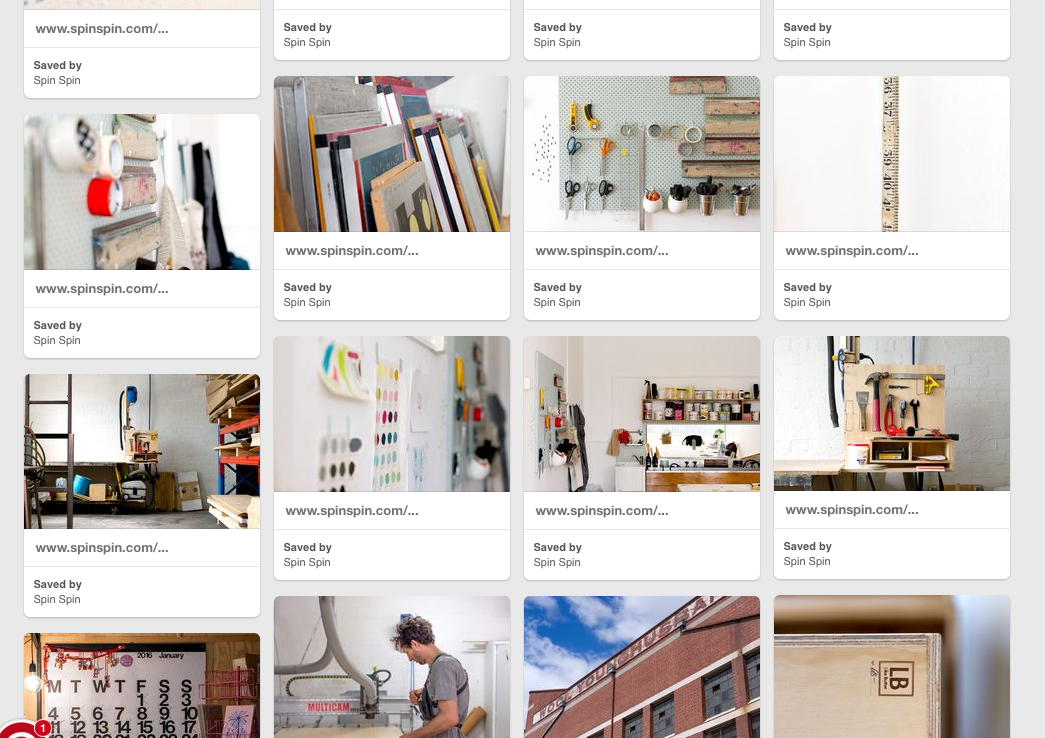The image showcases a curated selection of 12 similar craft-related products, arranged neatly within a square border. The layout features four items on top, four in the middle, and four at the bottom. Each product is accompanied by detailed information, including the website name and the individual who has saved the item, both of which are displayed in grey text below the product images.

The assortment includes various crafting materials and tools, highlighting items like wooden elements, a ruler, paint supplies, and hand tools such as a hammer and a wrench. Additionally, a calendar product can be spotted in the bottom left corner. The photographs of these products are exceptionally high quality, clearly showcasing the intricate details and craftsmanship of each item.